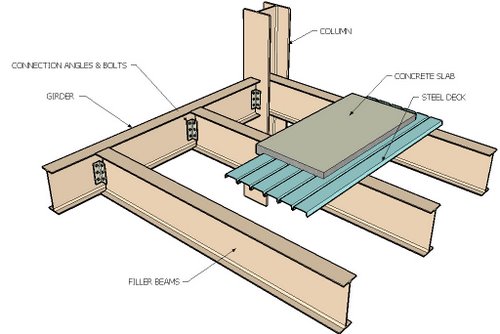The image is a detailed, color diagram of a steel frame construction, possibly for a building. Set against a white background with ample natural lighting, the image clearly showcases various structural elements with black arrows and text labels indicating each part. The steel frame features interconnected I-beams, including a vertical column in the center, and I-beams extending from both the left and right sides of the image. Additional I-beams are positioned perpendicularly to the central structure, with connection angles and bolts highlighted at key junctions. The diagram also shows a piece of light bluish-gray corrugated steel deck on the right side, topped by a rectangular gray concrete slab. Labels identify the girder, column, connection angles and bolts, filler beams, concrete slab, and steel deck, providing a comprehensive and detailed view of the construction elements. The overall color palette ranges from beige to olive green, enhancing the clarity and depth of the image.